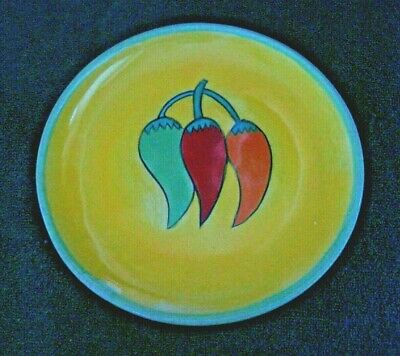The image depicts a yellow ceramic plate with a light blue border. The plate, which appears to be painted and glazed, has a reflective surface. In the center of the plate is a simplistic, children's-style illustration of three teardrop-shaped peppers connected at the stem. The peppers are arranged with a green pepper on the left, a red pepper in the middle, and an orange or yellow pepper on the right. The clean lines and minimal detailing of the illustration give it a charming, whimsical appearance. The plate is set against a dark navy blue background, and the image benefits from clear natural lighting that highlights the colors and glaze, even though the resolution is slightly low.